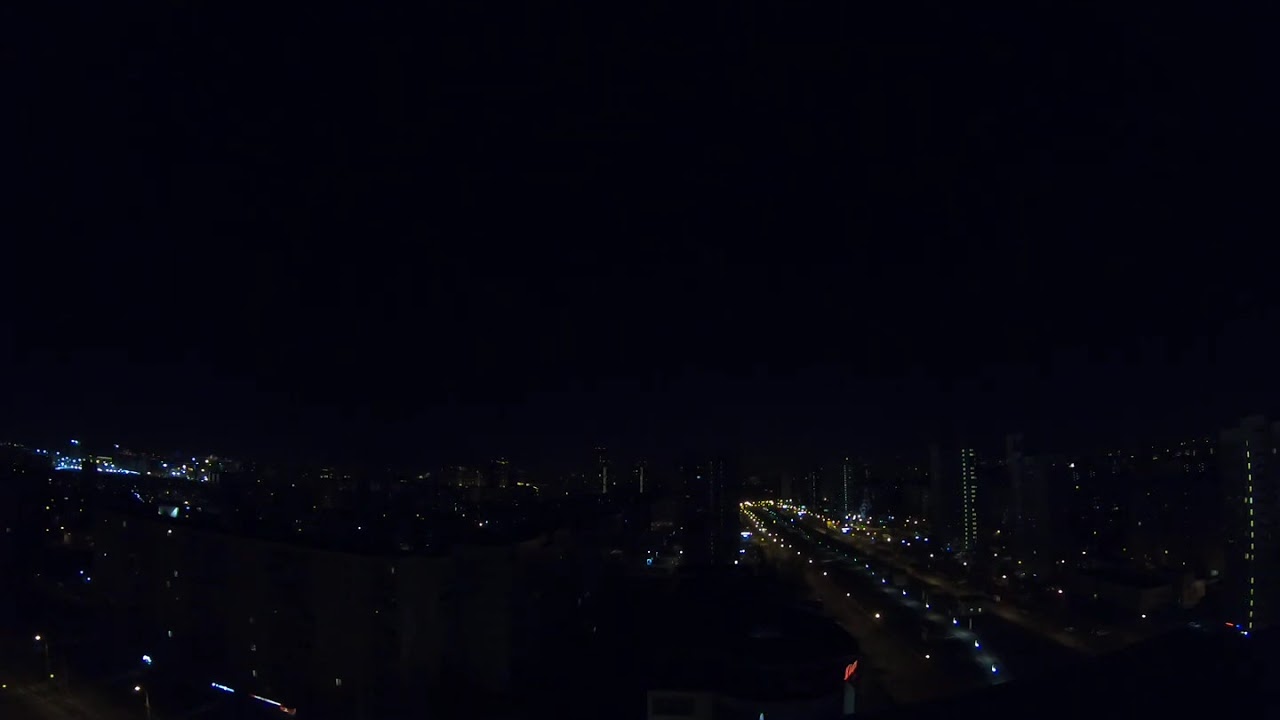This aerial photograph captures a cityscape at night under a cloudless, moonless black sky. The city below, prevalent in the bottom half of the image, is dominated by the right side where several high-rise residential buildings display long strips of lights, though most individual units remain dark. To their left lies a large, almost empty highway, illuminated by a mixture of white and yellow street lights, creating three distinct rows of lights stretching from the bottom right corner towards the center of the image. Adjacent to the highway on the left is a notably darker area with minimal lighting, rendering it nearly invisible. More distant structures with scattered lights can also be discerned further in the background.